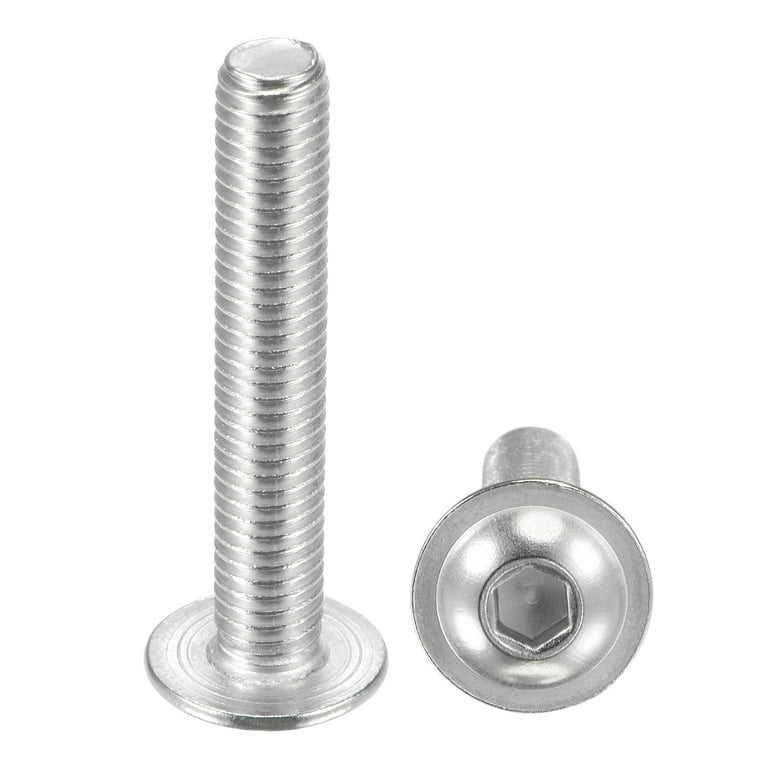The image features a close-up view of two machine bolts against a white background. On the left, a shiny, cylindrical bolt stands upright on its hexagonal head, with its threaded length extending vertically. The bolt is a bright silver color with distinct threads running up to its smooth end, creating a darker stripe along its highly reflective surface. On the right, a similar bolt lies horizontally, with its hex head facing the camera. The hex head features a hexagonal inlet, designed for an Allen wrench, with visible threads above the head. The bolts, possibly made of aluminum, are positioned on an empty, white surface, highlighting their metallic sheen and detailed texture.